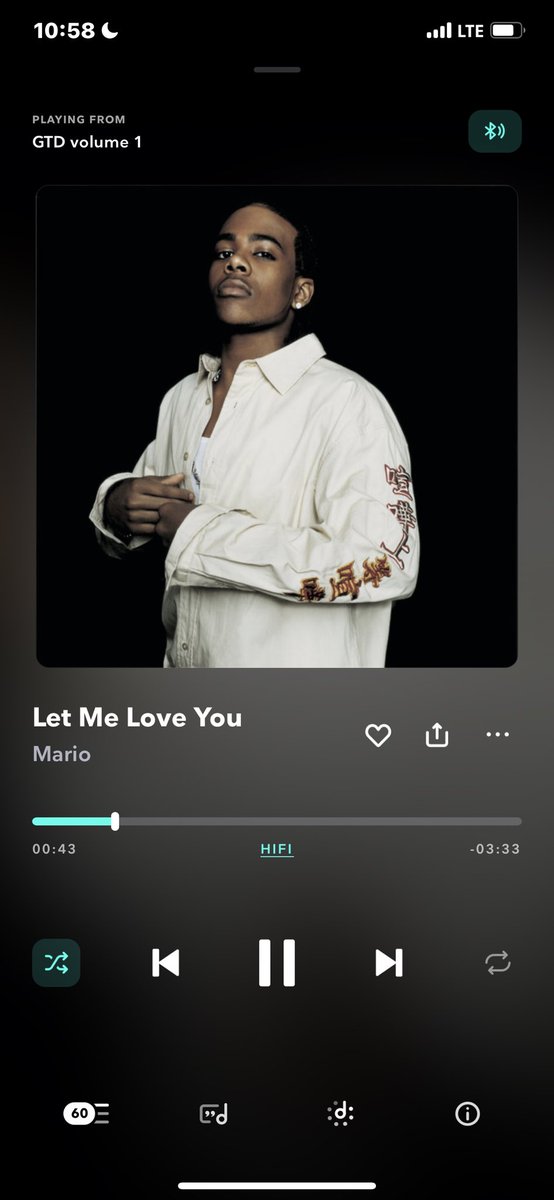The image displays a cell phone screen with a full battery and a strong LTE connection, indicated by multiple bars. The time is 10:58 AM, and the phone is set to "Do Not Disturb" mode. The screen is showing a music player with the song "Love Me, Love You" by the singer Mario. The track is already in progress, as indicated by a progress bar at the bottom. The left portion of the bar is teal green, showing the part of the song that has played, while the rest is gray. Beneath the progress bar, "Hi Fi" is written in teal. 

The album cover features a close-up image of Mario, who is an African American man looking upwards. He is wearing a white button-down shirt with a design running down one sleeve. His hands are cupped together in front of his chest.

Below the album art and progress bar are music control icons including pause, fast forward, reverse, and a box with crossed arrows, all highlighted in teal. Additionally, there are four other icons at the very bottom of the screen: one with the number 60, another resembling a letter 'D' inside a square box, a 'D' inside a circle, and a circle with an 'i' inside.